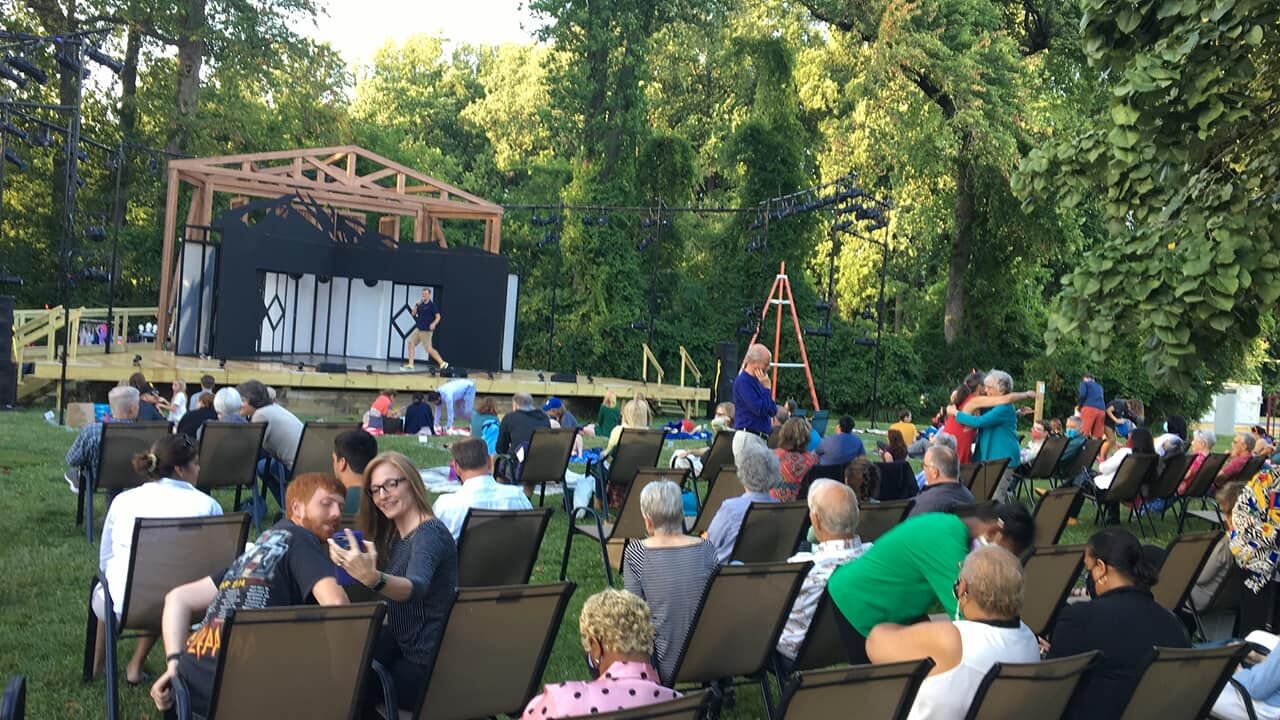The image captures the scene of an outdoor concert or performance in an open field surrounded by a dense area of trees. The event takes place on a sunny, warm day, as indicated by the attire of the audience members, who are mostly wearing just shirts. The stage itself is a plain, uncolored wooden structure with some cloth pieces hanging as part of the background decoration, adding a hint of black and white to the otherwise natural setup. On the stage, a person appears to be working, suggesting the performance has not yet begun.

In the foreground, a diverse audience of varying ages is seated on light brown lawn chairs, with some additional people sitting directly on the grass at the front. The crowd, numbering around 50 individuals, is engaged in different activities while they wait; some are taking selfies, others are standing, walking, or hugging. A few have masks on, hinting at a post-pandemic setting. The scene is vibrant with different colored shirts on the attendees, ranging from green to dark blue, light blue, and red. Overall, the setting exudes a relaxed, communal atmosphere against the backdrop of green grass and clear blue skies.